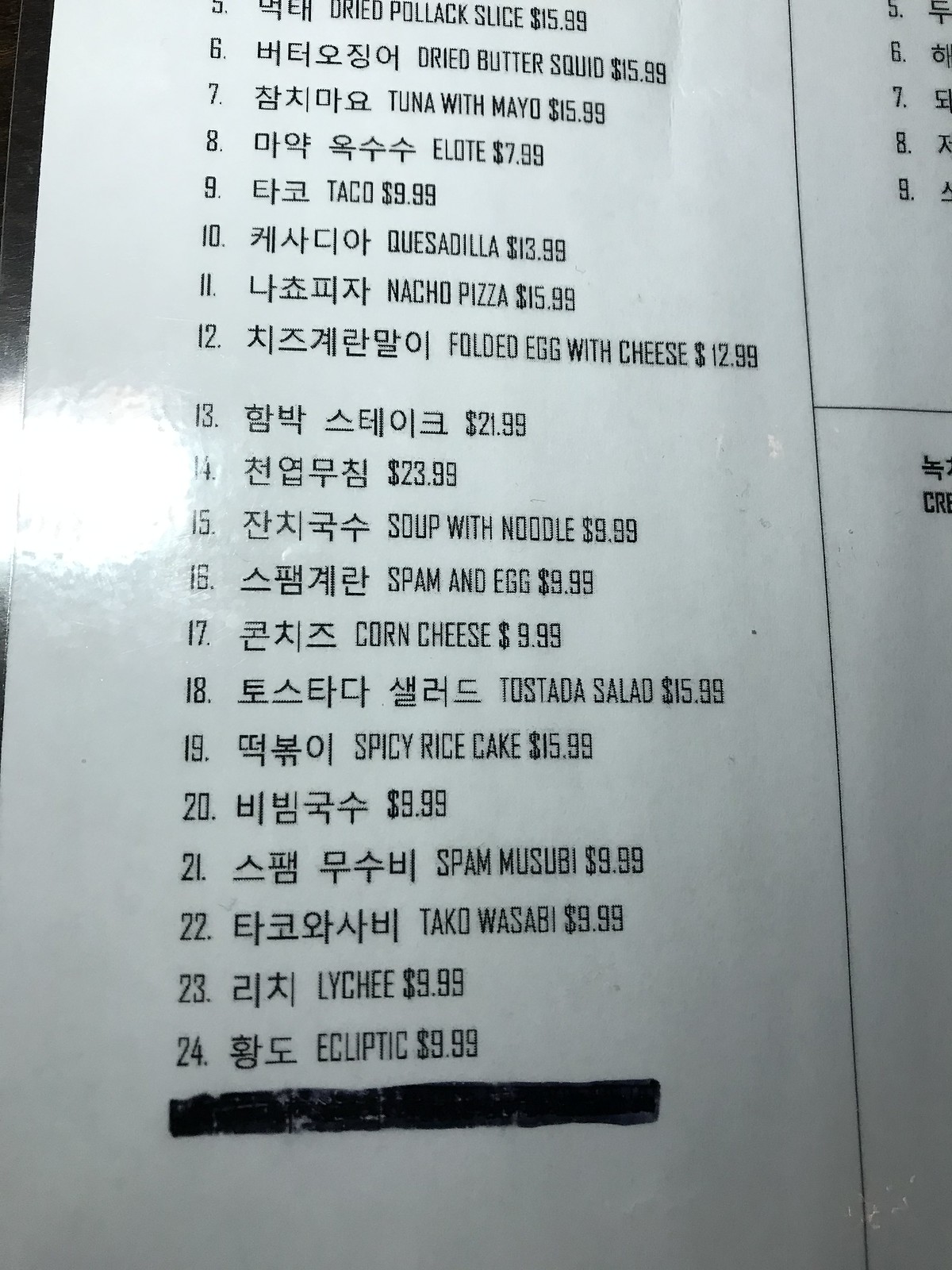In this detailed photo of a menu, we can't determine the exact name or location of the establishment. However, the bilingual text suggests that it is either a Korean restaurant or a place that offers Korean cuisine. The menu features a variety of dishes with prices listed in both Korean and English. 

Prominent items include:
- Dried Pollock Slice for $15.99
- Dried Butter Squid for $15.99
- Tuna with Mayo for $15.99
- Elope for $7.99
- Taco for $9.99
- Quesadillas for $13.99
- Nacho Pizza for $15.99
- Folded Egg with Cheese for $12.99

Some items are written only in Korean, indicating a possible language barrier for some patrons. Among the decipherable items, we also see:
- Soup with Noodles for $9.99
- Spam and Egg for $9.99
- Corn Cheese for $9.99
- Tostada Salad for $15.99
- Spicy Rice Cake for $15.99

Followed by another Korean-only item, the menu then lists:
- Spam Musubi for $9.99
- Taco Wasabi for $9.99
- Lychee for $9.99
- Ecliptic for $9.99

On the right-hand side, there are sections of the menu that are partially visible, but they are cropped out, leaving us with an incomplete view of all the offerings. The diversity in the menu options, from traditional Korean dishes to more eclectic fusion items, hints at a restaurant that embraces a mix of culinary influences.